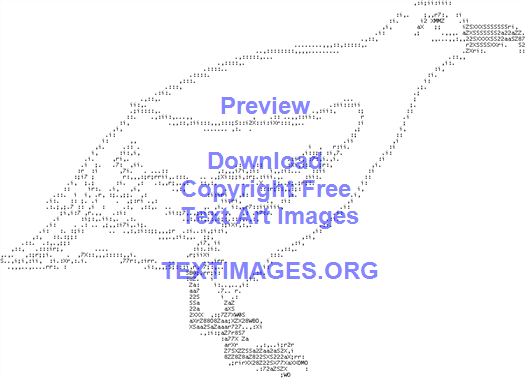The image depicts a detailed computer-generated side profile of a seagull, facing to the right on a clean white background. The seagull’s outline, comprising various numbers and letters, showcases distinct features including its beak, eye, wing, tail, and webbed feet, mimicking a dot matrix printer style. The body of the seagull remains unfilled, enhancing its distinctive shape. Above the artwork, in all capitalized, purple lettering, "PREVIEW, DOWNLOAD, COPYRIGHT FREE TEXTART IMAGES" is prominently displayed, followed by the website "textartimages.org". The lettering also appears blue in some accounts. The overall composition highlights the bird made entirely from text characters, emphasizing its unique form and detail.